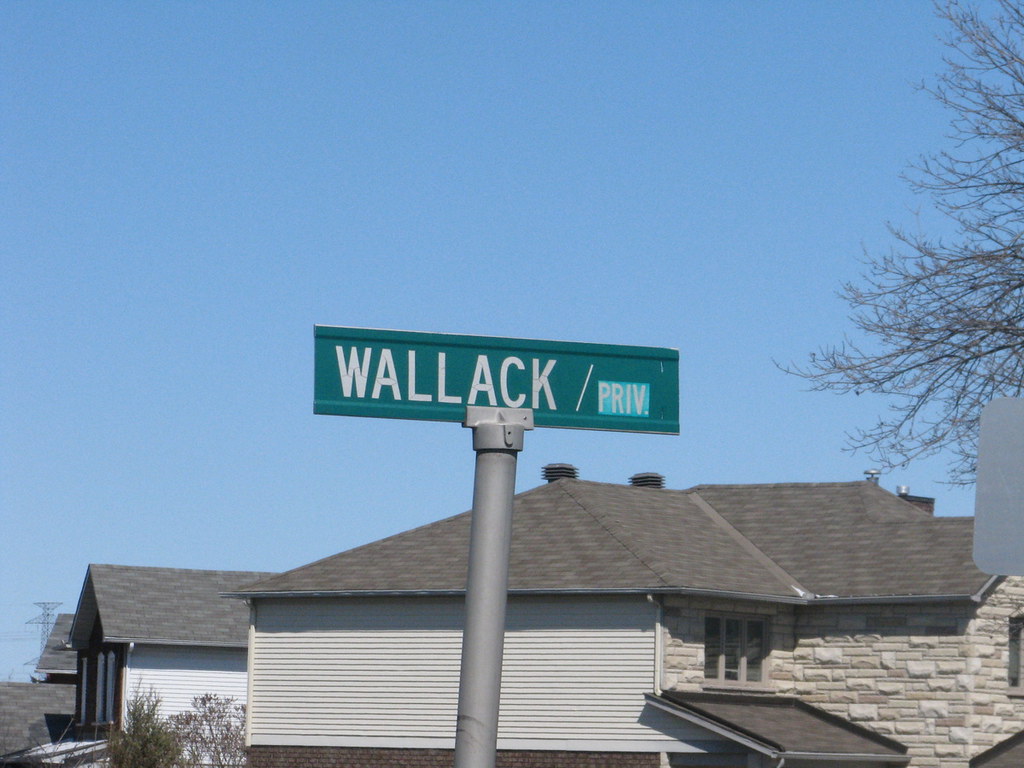The photograph features a prominent green street sign with bold white lettering, displaying "WALLACK" with "PVT" slashed diagonally across, indicating a private area. The sign is mounted on a metal post. In the background, an array of elegant homes with stone facades and brown shingle roofs can be observed. One house stands out in the immediate vicinity, showcasing its refined architectural details. The backdrop reveals a clear blue sky without any clouds, and a leafless tree suggests that the season is winter.